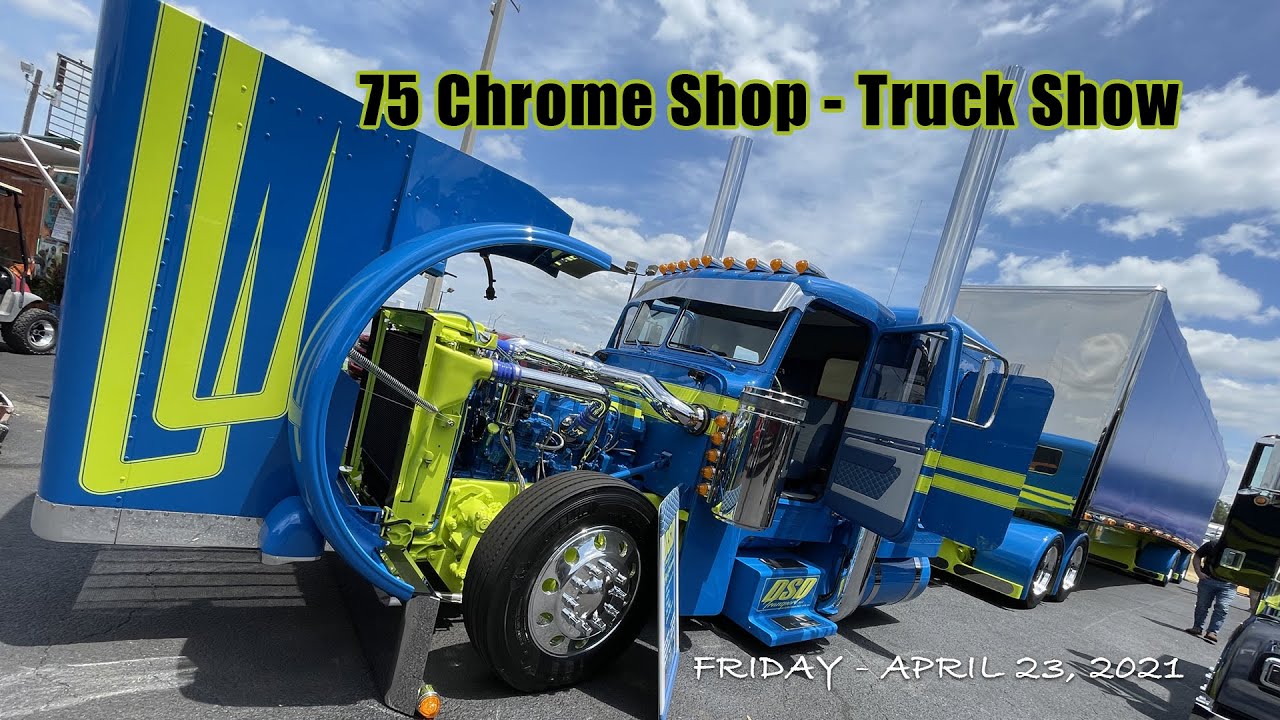This advertisement for the 75 Chrome Shop Truck Show, scheduled for Friday, April 23, 2021, depicts a meticulously detailed and custom-painted semi-truck against a backdrop of a bright blue, cloud-filled sky. The truck, the main attraction, is an 18-wheeler with an electric blue cab featuring double doors that open outward in reverse fashion. Vibrant lime green or fluorescent yellow trim accents the hood, front fenders, and stripes along the side and door. The highly polished cab includes gleaming chrome details on the rims, protruding lug nuts, mirrors, and brackets. The hood is lifted to reveal the blue engine with visible silver pipes and components, highlighted by a yellow radiator. The truck's roof features orange lights and a silver visor, complemented by two standing silver exhaust pipes. A reflective silver trailer, likely a soft-sided trailer with a gray cover rather than actual chrome, elongates the truck's impressive length. The scene unfolds on a concrete road with spectators on the ground, including a man with his arm on his hip observing the truck. The image is structured with the event title in black print and green-bordered letters at the top, while the date is noted in white letters at the bottom right.